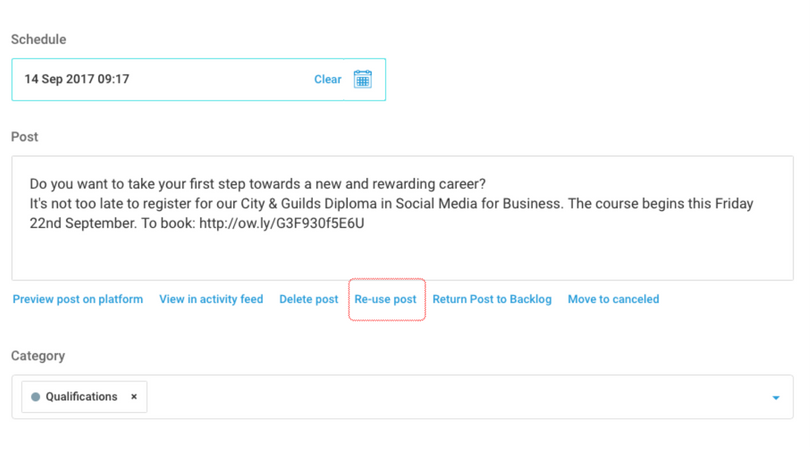The image features a predominantly white background with light black text at the top, displaying the word "Schedule" with a capitalized "X". Below this, there is a blue-green trim that contains the date "14 September 2017" formatted as "09/17". 

Further down, in blue print, the word "Clear" is depicted alongside a calendar graphic. Beneath this, the text "Post" is shown in the same gray print color with a capital "P". Within a gray, thin-outlined box, it reads: "Do you want to take your first step towards a new and rewarding career? It's not too late to register for our City and Guides Diploma in Social Media for Business. The course begins this Friday, 22nd September. To book: http://ow.ly/G3F930F5E6U."

Exiting the outlined box, the image contains several options in blue print: "Preview Post on Platform," "View Inactive Activity Feed," "Delete Post," "Reuse Post," and "Return Post to Backlog," with "Reuse Post" enclosed in a red square.

Finally, the image labels the "Category" section with a dropdown menu where "Qualifications" is selected, accompanied by an "X" next to it.